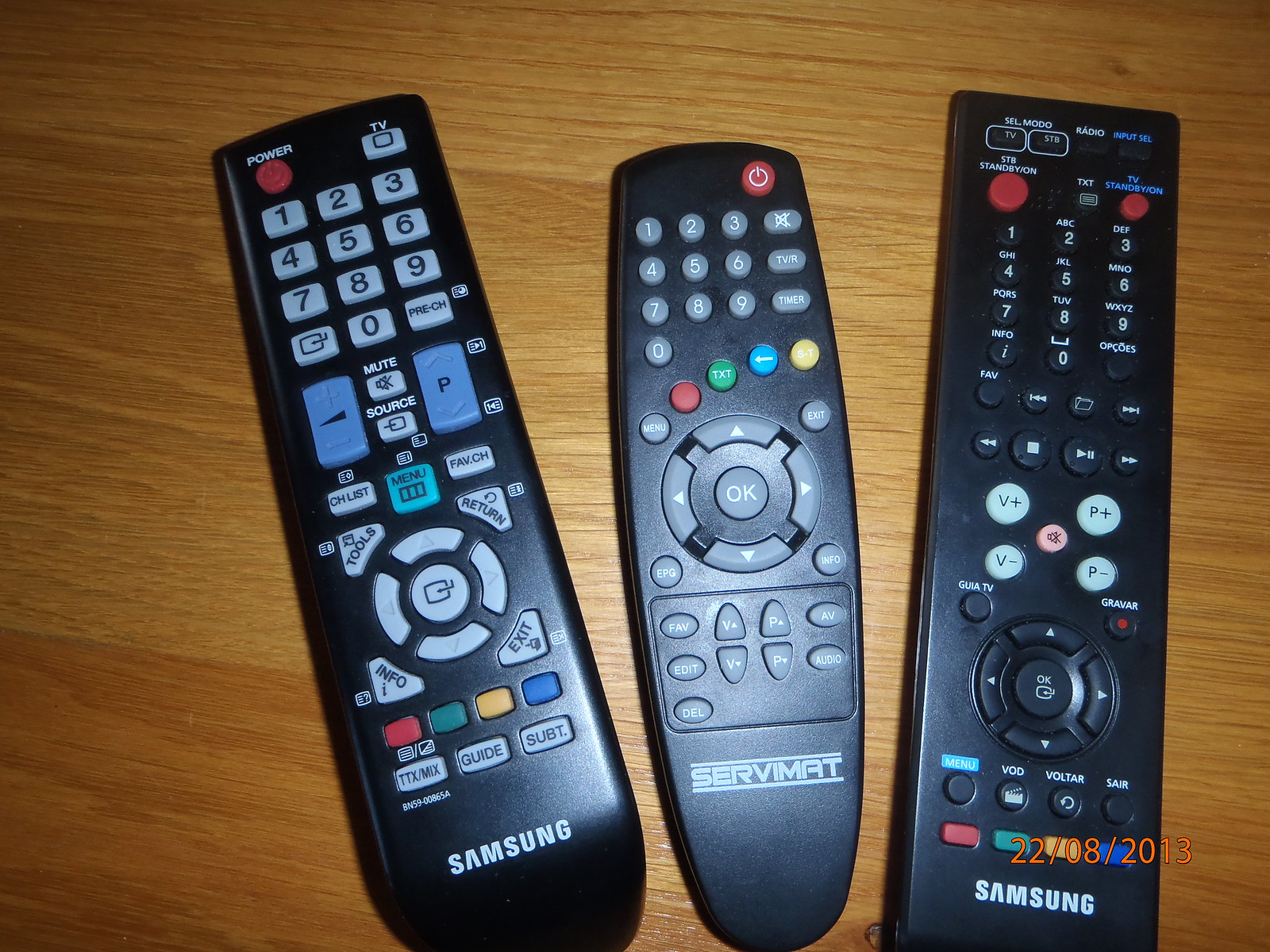This color photograph, dated 22/08/2013 in orange text situated in the bottom right corner, captures a view looking directly down onto three remote controls laid on a wooden, grainy surface. The wooden surface displays variations in tone, with darker shades toward the bottom left and lighter tones at the top, and features grain running horizontally across the image. Each remote is black plastic with an array of buttons, positioned in a line from left to right.

The first remote on the left, branded Samsung, is rectangular with a rounded bottom. It features an assortment of buttons including directional keys, numbers, and four colored buttons (red, green, yellow, blue) near the bottom. 

The middle remote, marked ServiMAT, is narrower, with a more pronounced taper at the bottom and a slightly rounded top. It includes numerous buttons and a prominent "OK" button at its center.

The remote on the right, also a Samsung, is the largest. It shares a similar rectangular shape with the left remote but has a slightly different button configuration, including directional keys, numbers, and additional electronic control functions.

Together, these remotes illustrate the design variations and standard functions typical of television or multi-device controls from the early 2010s, a reflection of the period's technology.